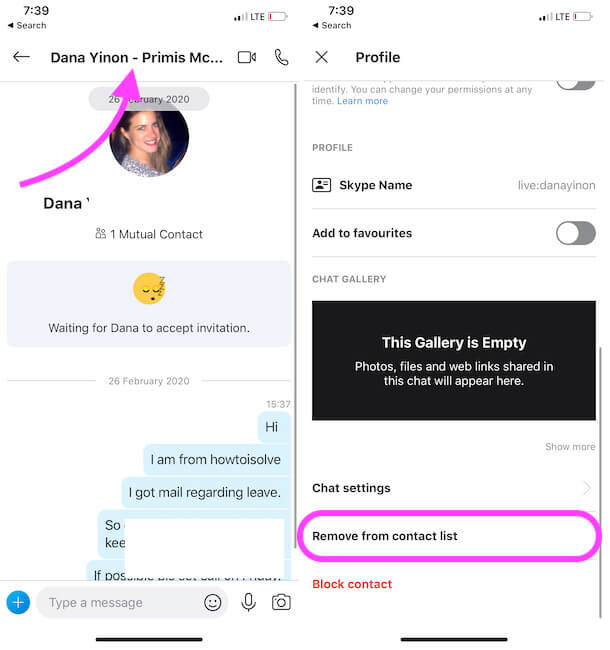A set of two side-by-side cell phone screenshots is displayed. The screenshot on the left showcases a profile named "Dana Ynon," with a highlighted minus sign indicated by a purple arrow next to the name. Below the name is Dana's profile picture, followed by the text "1 mutual contact." Just beneath that, it indicates "Waiting for Dana to accept the invitation." Further down, there's an additional text that isn't specified. The screenshot on the right depicts a Skype profile page with "Skype Name," stating "live.danayinon."